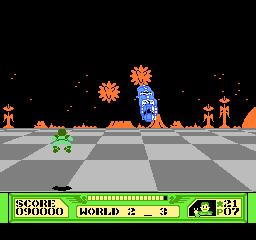This image captures a scene reminiscent of an 1980s arcade game. The foreground displays a classic video game interface with a green ribbon banner at the bottom, segmented with yellow sections, bearing the text "Score: 90,000." Additionally, it shows "World 2_3," alongside an icon of a character and the notation "*21P07," which might indicate player 7.

The scene unfolds in a cosmic setting, with a checkerboard landscape floating in the blackness of space adorned with twinkling stars. A small green character is depicted jumping across the checkerboard squares. In the distance loom green and orange mountain-like structures or possibly spaceships, enhancing the retro sci-fi atmosphere. Furthermore, a blue object sits vaguely in the far background, adding to the intricate, nostalgic visuals typical of classic arcade games.